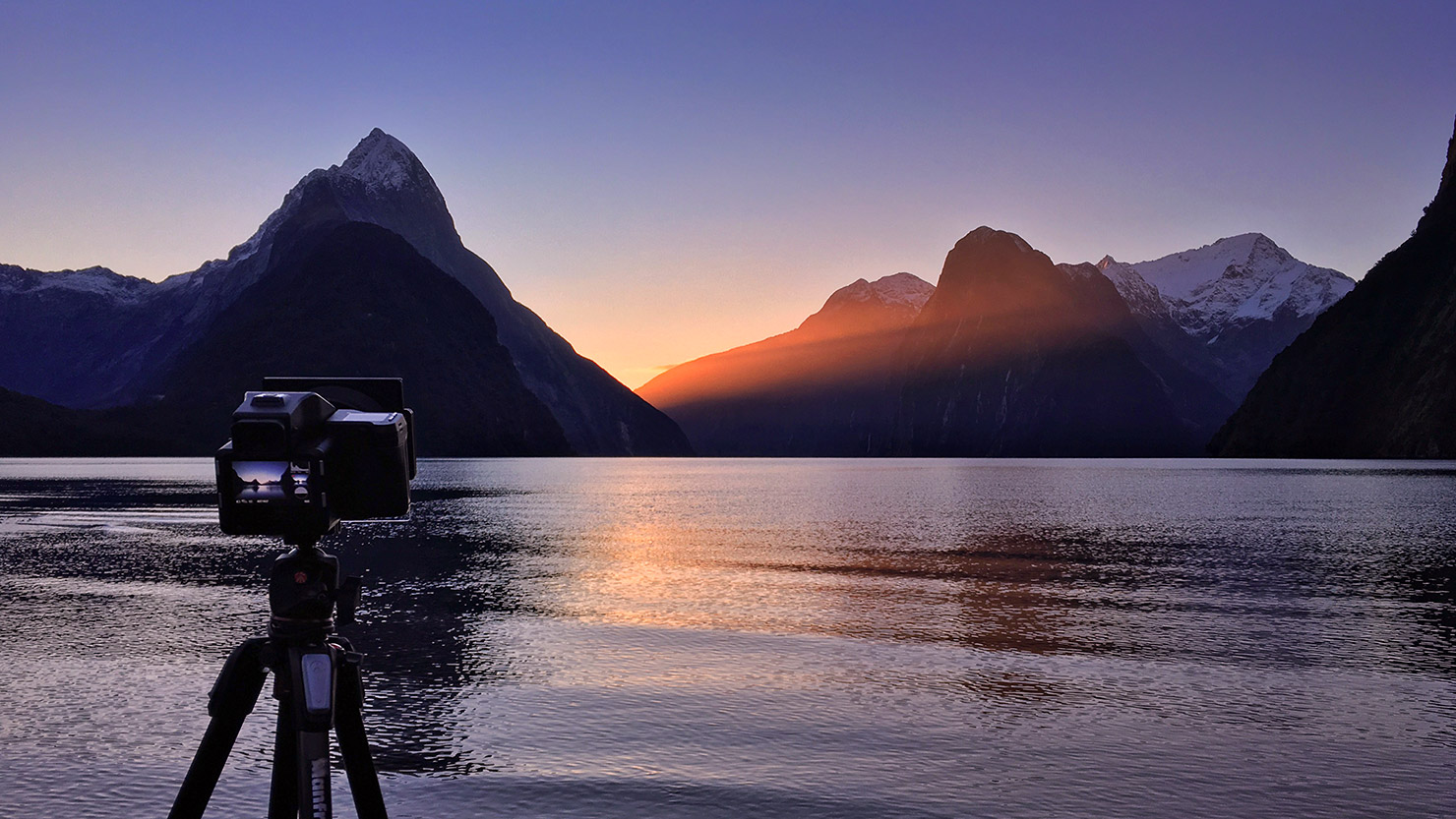The image features a serene, realistic-looking landscape that evokes a sense of tranquility. Set either at dawn or dusk, the overall tone is a muted blue, contrasting with the warm orange hue of the sunlight peeking through a deep valley between towering mountain ridges. A wide, calm body of water—whether a lake or the ocean—spans the foreground, leading the eye towards the high mountain range that descends down to the water's edge. In the lower left corner of the frame, a camera mounted on a tripod is set up, aiming towards the breathtaking scene where the mountains frame the emerging sunlight. The composition captures the quiet beauty of nature, with an emphasis on the interplay of light and shadow across the landscape, highlighting the beginning or end of the day.